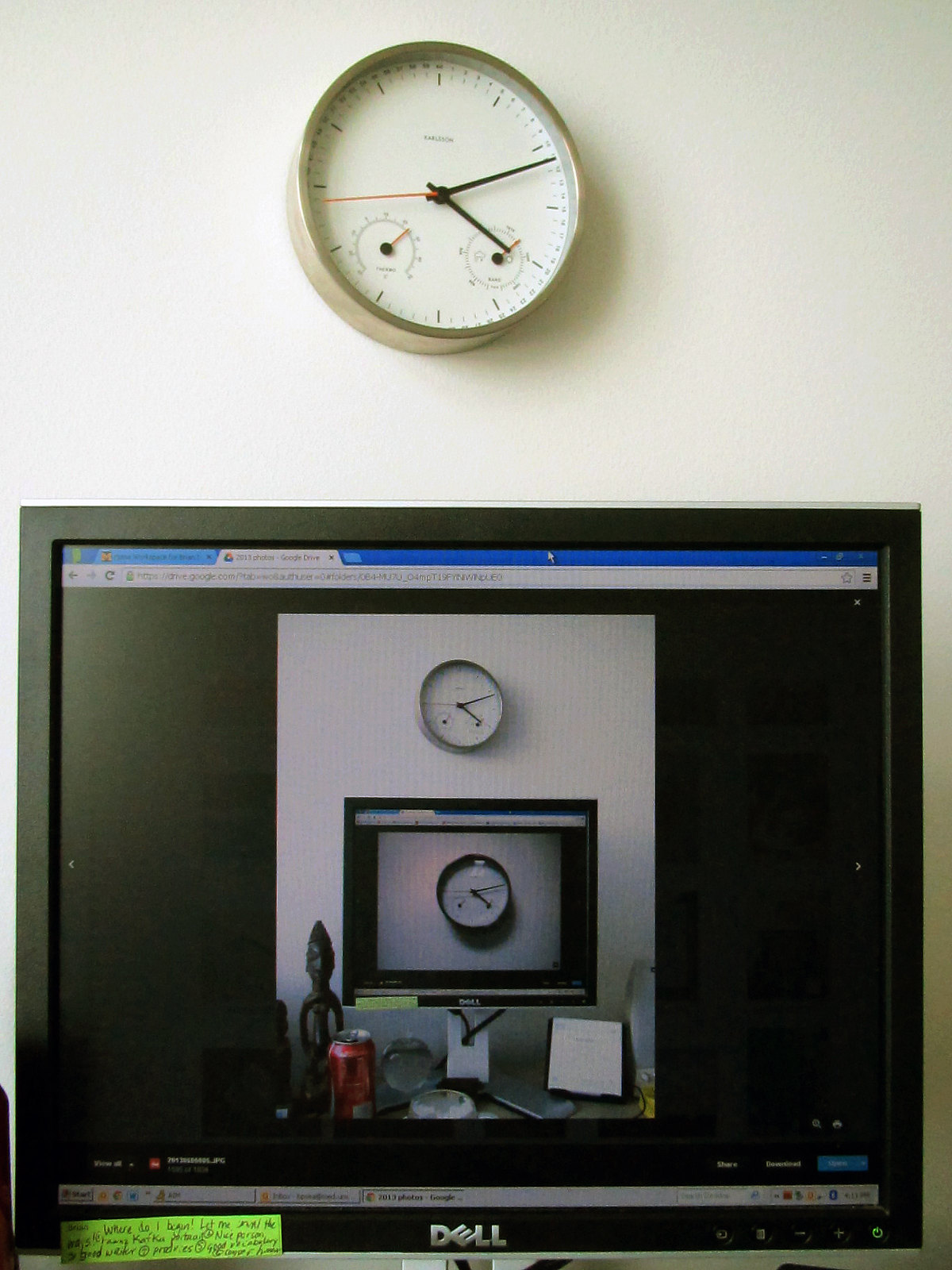The photograph captures a detailed scene of a cluttered office desk with a close-up of a Dell computer monitor. Situated against a plain white wall, the monitor displays an image that recursively shows itself in a seemingly infinite cascade. Mounted on the wall above the monitor is a simplistic wall clock with black hands pointing to approximately 4:10, featuring a silver or gold rim and a pair of gauges at the bottom; the clock face is devoid of numbers, substituting small dashes instead. The monitor, characterized by its thick black border and black screen background, reveals mostly black content with the entire scene mirrored within its display. A neon green Post-it note is affixed to the bottom left of the monitor, displaying three lines of text that begin with "Where do I begin, let me count the ways," although the rest becomes difficult to decipher. The setup, filled with these recursive visuals and the small personal touch in the form of the sticky note, portrays a snapshot of an everyday office environment.